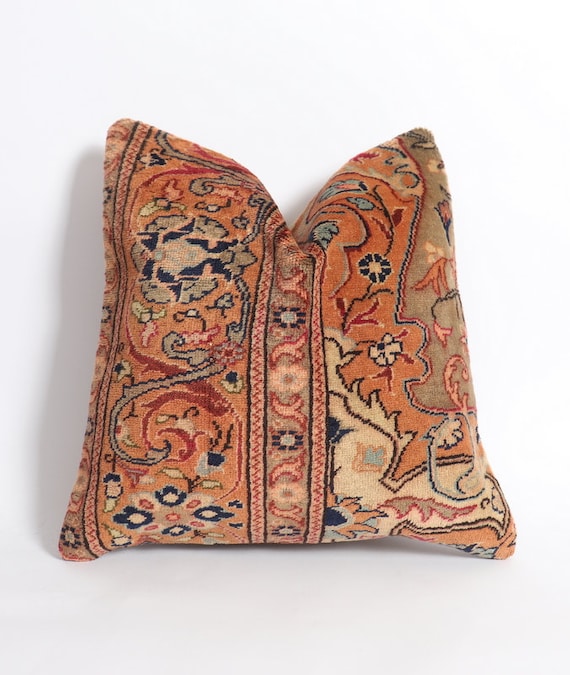This image features an old, square-shaped throw pillow with a noticeable divot at the top, lying on a stark white background which accentuates the pillow's details. The pillow, possibly hand-stitched, showcases a predominantly light orange and tan fabric with a varied pattern that exudes a vintage, possibly Southwestern or African-inspired aesthetic. Its intricate design displays multiple floral motifs and an abstract arrangement, including elements resembling flowers, stars, and vertical lines with orange squiggles. The color palette is dominated by orange, interspersed with sparse patches of blue, white, black, beige, brownish-green, and red. Notably, a band with a floral motif runs across the middle, enhancing the handcrafted feel. The photograph focuses solely on the pillow, capturing its shadow on the left side and slightly on the upper top, perhaps intending to highlight the pillow's unique characteristics for potential sale on platforms like eBay or Etsy.